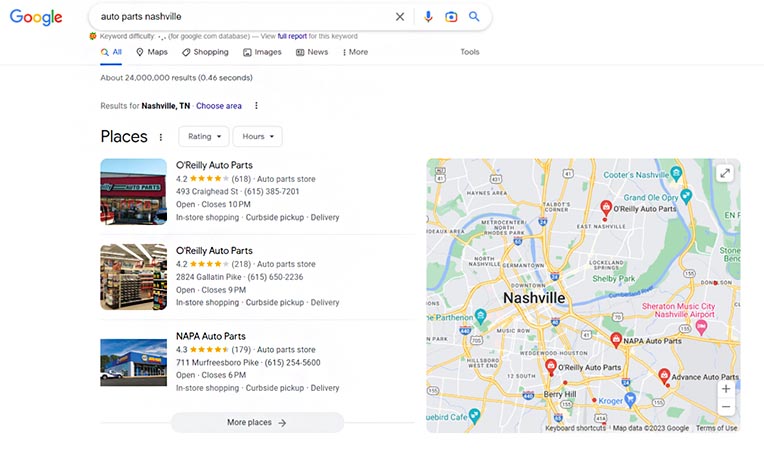The image depicts Google search results for the query "auto parts Nashville." In the upper left corner, the iconic multicolored Google logo is prominently displayed. Dominating the top of the page is the search bar, with the entered query clearly visible. Directly below the search bar is the menu strip, offering options such as All, Maps, Shopping, Images, News, and More.

The focus of the search results is on locations identified as "Places" for auto parts stores in Nashville, Tennessee. The first two results are for different branches of O'Reilly Auto Parts, each accompanied by a photograph on the left and a brief description. Following these is a listing for Napa Auto Parts, similarly illustrated with an image and description. 

At the bottom of these local listings, a gray button labeled "More places" invites further exploration. To the right of the page, a map visualizes the search results with multiple red teardrop markers indicating the locations of various auto parts stores throughout Nashville.